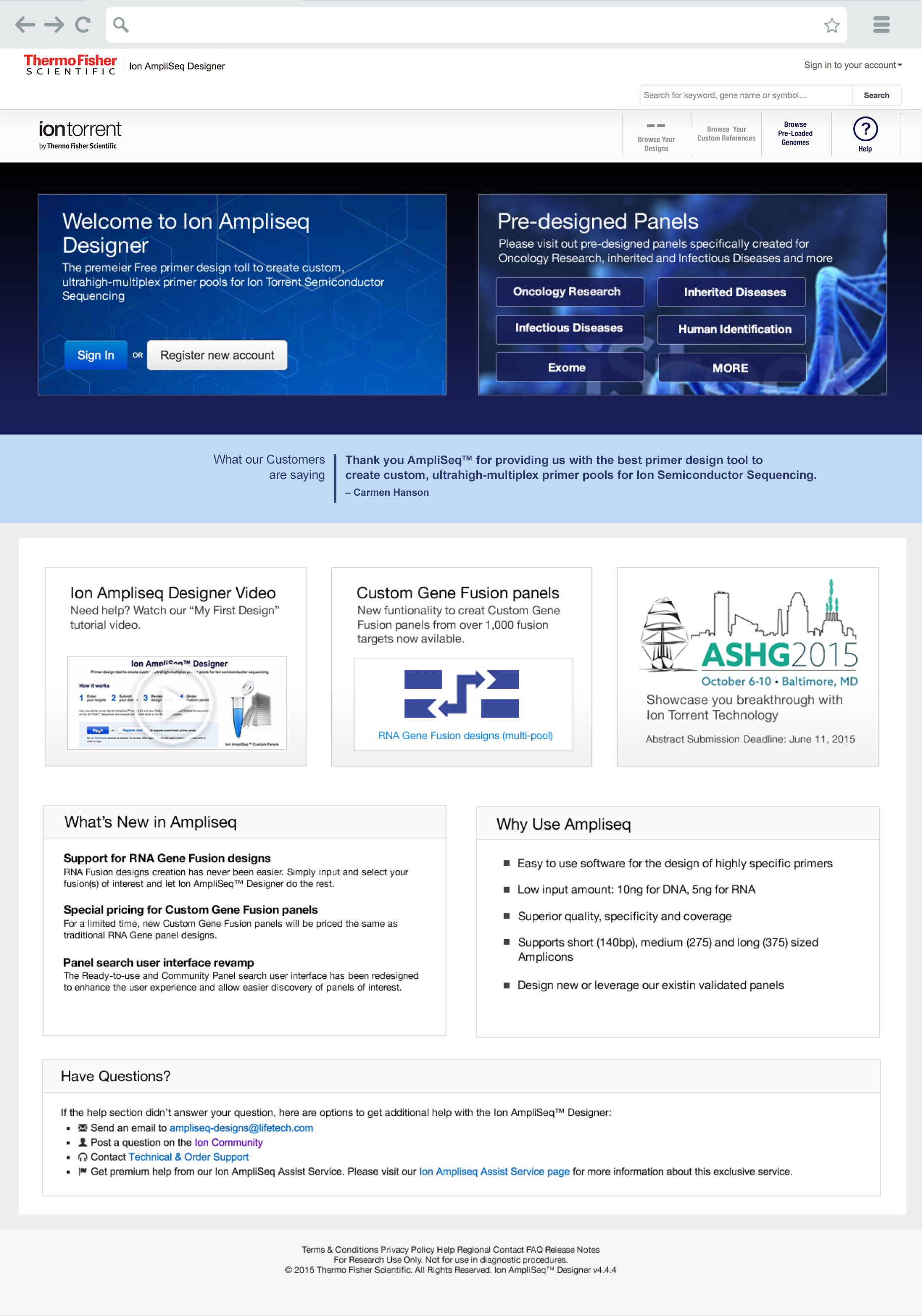Screenshot of the Thermo Fisher Scientific website interface. At the top of the page, a gray navigation bar features standard browser controls: back and forward arrows, a refresh icon, a star icon for bookmarking, a search bar, and a menu option on the far right. Below this is a white bar displaying the Thermo Fisher Scientific logo on the left, with a sign-in prompt for user accounts on the right.

The next layer is a gradient bar that transitions from white at the bottom to tan at the top. This bar contains the header "Ion Torrent" in black lettering on the left, alongside navigation options on the right, including a help link.

The central portion of the screenshot displays information about the "Ion AmpliSeq Designer" against a blue to black gradient background. A pre-designed panel selector is featured prominently, with a zoomed-in visual of blue DNA strands overlaying the top of the background.

One bar down, a light blue section highlights customer testimonials under the heading "What Our Customers Are Saying."

At the bottom of the screenshot, a white square contains infographics detailing the latest updates and features of the Ion AmpliSeq Designer, including its uses and advantages, along with links to frequently asked questions.

The detailed composition of the webpage provides a comprehensive overview of the various sections and functionalities, enhancing user navigation and information accessibility on the Thermo Fisher Scientific website.